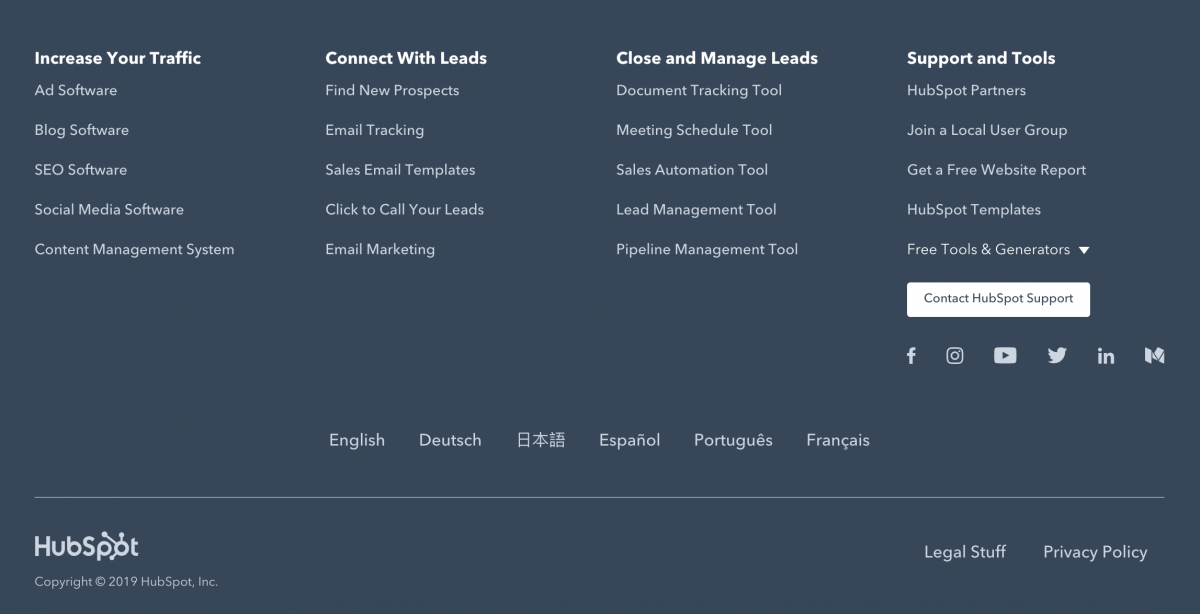The image depicts the footer section of the HubSpot website, dated 2019, providing various functionalities and information. The footer is organized into four primary columns under distinct headings, filled with useful links for users.

- **Bottom Bar Information**:
  - **Copyright**: 2019, HubSpot Inc.
  - **Languages Available**: English, German, Japanese, Spanish, Portuguese, French
  - **Legal and Privacy Links**: Includes legal information and privacy policy
 
- **Column 1: Increase your Traffic**:
  - **Links Included**: 
    - Add Software
    - Blog Software
    - SEO Software
    - Social Media Software
    - Content Management System

- **Column 2: Connect with Leads**:
  - **Links Included**:
    - Find New Prospects
    - Email Tracking
    - Sales Email Templates
    - Click to Call Your Leads
    - Email Marketing

- **Column 3: Close and Manage Leads**:
  - **Links Included**:
    - Document Tracking Tool
    - Meeting Schedule Tool
    - Sales Automation Tool
    - Land Management Tool
    - Pipeline Management Tool

- **Column 4: Support and Tools**:
  - **Links Included**:
    - HubSpot Partners
    - Join a Local User Group
    - Get a Free Website Report
    - HubSpot Templates
    - Free Tools and Generators